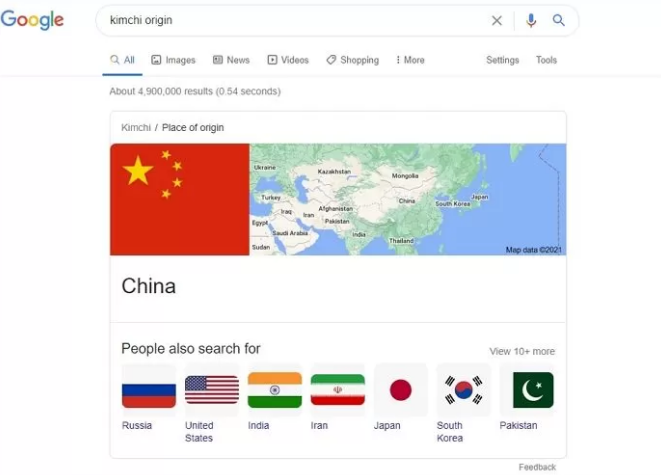In the image, the top left-hand corner features the Google logo followed by the familiar Google search bar. Within the search bar, the query "Kim Chi origin" is entered. According to the main search results, there are approximately 4,900,000 results, and the search took 0.54 seconds to complete. 

Prominently displayed is the information stating that the origin of Kim Chi is China. Located just below this text, but above the word "China," there is an image of the Chinese flag. To the right, there is a topographical map highlighting the geographical location of China. 

Below the main result, there's a section indicating that people also search for "Russia, United States, India, Iran, Japan, South Korea, and Pakistan." Each of these countries is represented with their respective national flags shown above the list. There is also an option to view more related searches above this section.